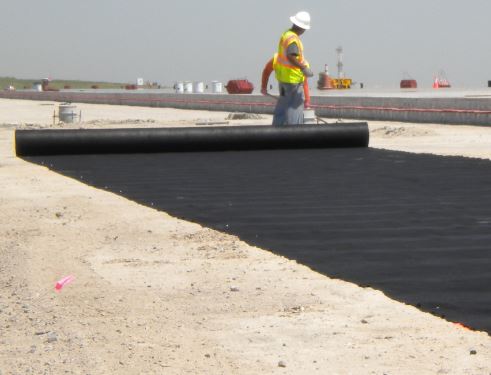In this image, we see a construction site set against a dark and cloudy sky, suggesting imminent rain. Prominent in the foreground is a gentleman clad in a yellow and orange safety vest and a white hard hat, standing on what appears to be a large black mat unrolled over sandy terrain. Just in front of him, another worker in an orange shirt is engaged in ground work. Scattered around the site are various grains and rocks, adding to the rough texture of the area. Machinery, colored in red and orange, is visible in the background, hinting at ongoing construction activities. A notable feature is a small pink object, possibly a flag or marker, protruding from the ground in the bottom left corner of the image. Towards the horizon, subtle hints of a road or concrete pad can be seen, along with what might be a gas platform and some white drums, with a faint green hill on the far left edge of the scene. The overall impression is one of a busy construction site, meticulously organized amid challenging weather conditions.